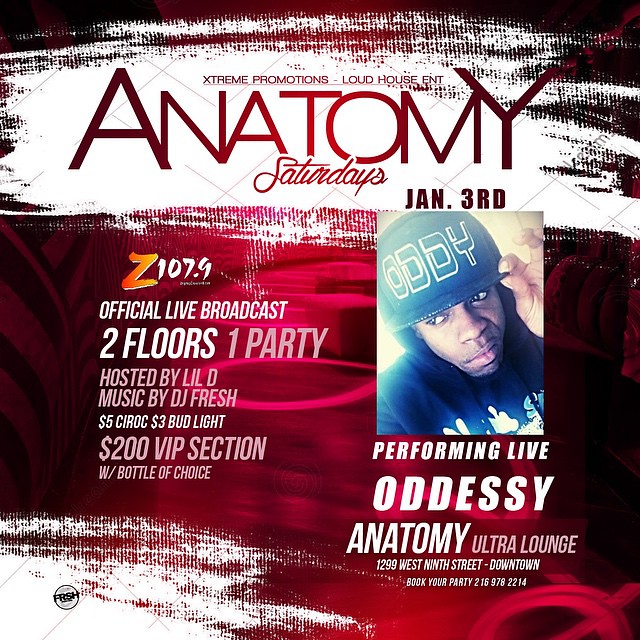The image appears to be a detailed advertisement flyer for a nightclub event at Anatomy Ultra Lounge. The background features a red and black theme with swirling neon and psychedelic lights, accentuated by a white swoosh across the top. At the center, large text announces "Extreme Promotions, Wild House Entertainment, Anatomy Saturdays." A key focal point is the photograph of a young African American man wearing a black baseball cap emblazoned with "O-D-D-Y" and a black sweatshirt. Below his image, text states "Performing Live: Odyssey," and specifies the event will be held on January 3rd at Anatomy Ultra Lounge, located at 1299 West 9th Street, Downtown. Additional promotional details include a live broadcast by Z107.9, with the event hosted by Lil D and music by DJ Fresh. Furthermore, enticing offers such as $5 Ciroc, $3 Bud Light, and a $200 VIP section with bottle service are highlighted to attract party-goers. The flyer serves to book parties with a provided contact number, enhancing its comprehensive advertisement appeal.